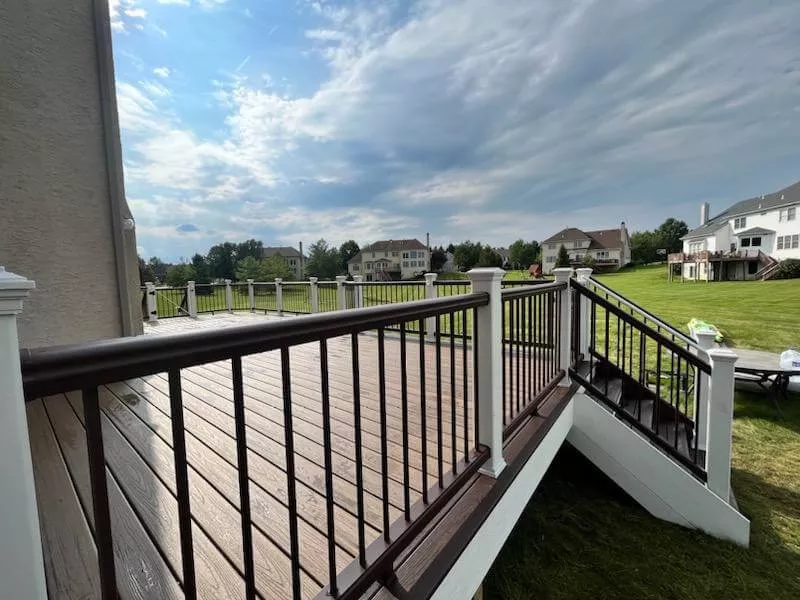This image captures a stunning view from the vantage point of an elegant mahogany deck, belonging to one of the multi-story homes in an upscale housing development. The deck features brown synthetic flooring and white-trimmed railings, complemented by stairs that descend to a large, lush, green common lawn area shared by similarly luxurious houses. These expansive homes, each approximately 4,000 to 5,000 square feet, boast multiple stories, large decks, numerous windows, and chimneys. In the background, a picturesque scene with tree-lined areas gives way to a partly cloudy sky, allowing patches of blue to peek through. The overall impression is one of sophistication and community, reminiscent of a high-end neighborhood that could be located in a scenic area like Florida or Georgia.